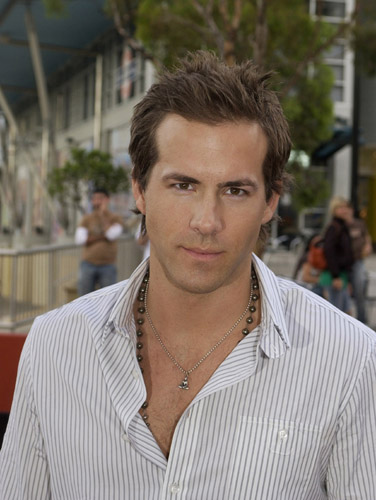The photograph captures actor Ryan Reynolds in an outdoor setting, seemingly in the middle of the day. Positioned centrally in the image, Ryan stands out with his attentive gaze directly into the camera. He sport a white button-down shirt adorned with fine pinstripes, with the top two or three buttons undone, revealing his chest hair and two necklaces: one a beaded, longer necklace and the other a smaller chain necklace with an indistinct pendant. His hair is styled with a noticeable lift at the front. The background is an urban area featuring a large building extending diagonally toward the upper left corner. Among the busy surroundings, several people can be seen walking, a few appearing blurry. A man with folded hands and additional pedestrians to the right add to the lively scene, along with trees and a street nearby, completing the composition.